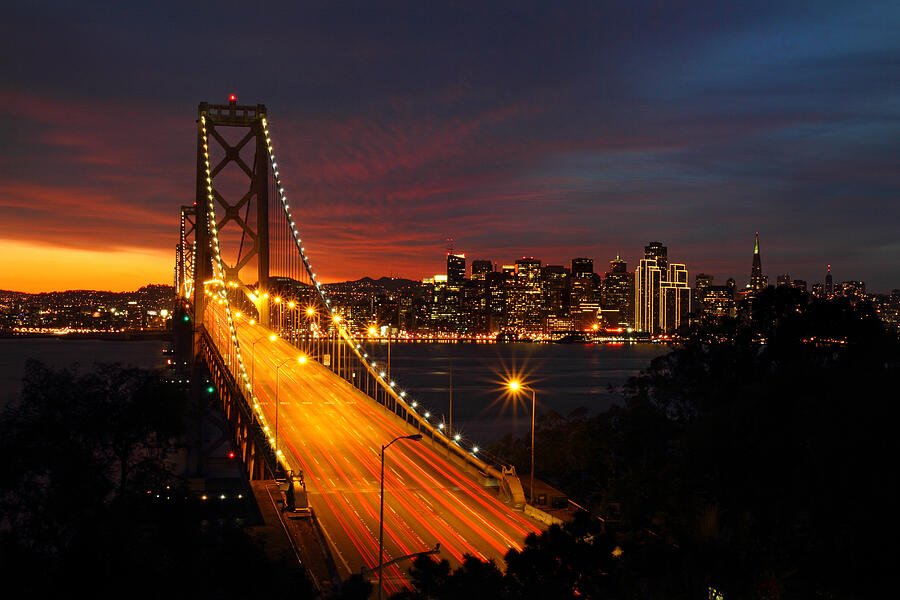A stunning nighttime cityscape captures the moment just after sunset, where the sky immerses in varying hues of grayish blue, red, and glowing orange near the horizon, accentuating the remnants of daylight. In the lower left-hand corner, the sun sets behind rugged mountainous terrain, casting a warm orange glow across the scene. The centerpiece of the image is a grand suspension bridge extending from the foreground into the distant city skyline, spanning a vast body of water. The bridge, adorned with lights along its entire structure and atop its suspenders, appears void of vehicles but shows streaks of light, adding an element of dynamism. In the backdrop, the city's tall buildings illuminate the night, their countless lights shimmering across the waters beneath and accentuating the intricate steel framework of the bridge. The overall atmosphere is a blend of twilight serenity and urban vibrance, presenting a harmonious juxtaposition of natural beauty and architectural grandeur.